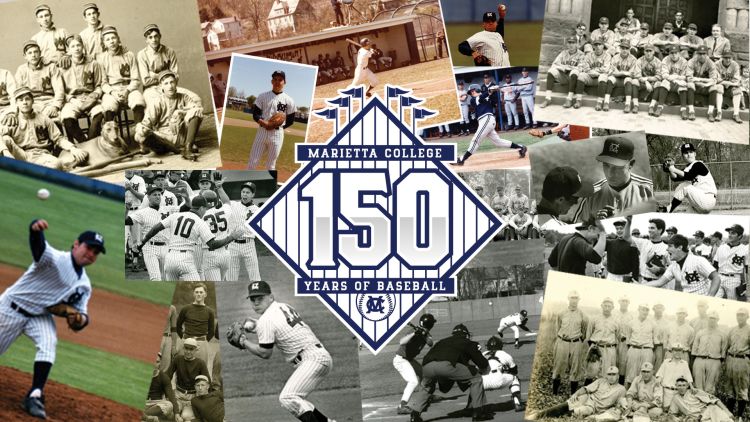This commemorative poster showcases a rich collage of photographs highlighting 150 years of baseball at Marietta College. At the center of the poster is a blue diamond logo with symmetrical sides, featuring the large text "150" and the Marietta College logo beneath. The title, "Marietta College, 150 Years of Baseball," frames the logo, with a baseball adorned with the "MC" insignia below. Surrounding the central emblem is an array of black and white and color photographs that chronicle the storied history of the college's baseball program. The images vary in size and depict diverse scenes, including team rosters, individual portraits, and action shots of players pitching, hitting, and fielding. The older photographs, primarily black and white, capture full team photos and remarkably historical moments, while the newer, color images likely date from the 1990s and more recent years. Accentuating the design are pinstripe vertical lines leading up to flag pennants, adding a nostalgic touch to the poster.